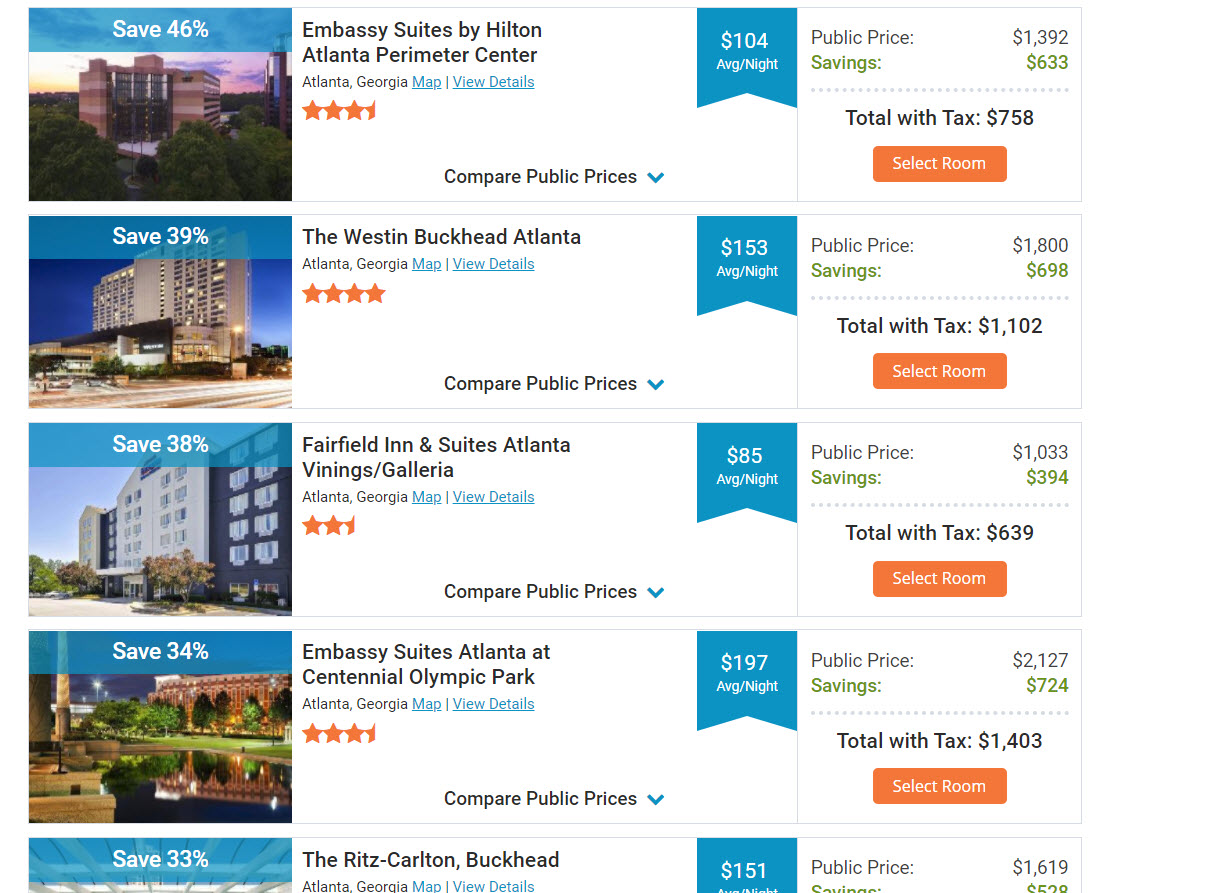On a white background, the image features a list of hotel listings, arranged vertically. Each listing is structured with a photo of the hotel on the left, details about the hotel in the middle, and pricing information on the right. The image displays four complete listings and one partial listing, each offering significant discounts.

1. **Embassy Suites by Hilton, Atlanta Perimeter Center, Atlanta, Georgia**:
   - **Discount**: Save 46%
   - **Map Details**: Included
   - **Average Price per Night**: $104
   - **Public Price**: $1,392
   - **Savings**: $633
   - **Total with Tax**: $758
   - **Button**: An orange "Select Room" button is prominently displayed.

2. **The Westin Buckhead, Atlanta, Georgia**:
   - **Discount**: Save 39%
   - **Average Price per Night**: $153
   - **Public Price**: $1,800
   - **Savings**: $698
   - **Total with Tax**: $1,102

3. **Fairfield Inn & Suites, Atlanta Vinings-Galleria**:
   - **Discount**: Save 38%
   - **Average Price per Night**: $85

Additional details for the remaining listings are partially visible, reinforcing the structured and comprehensive presentation of hotel options including images, average nightly rates, savings percentages, and total costs with taxes.